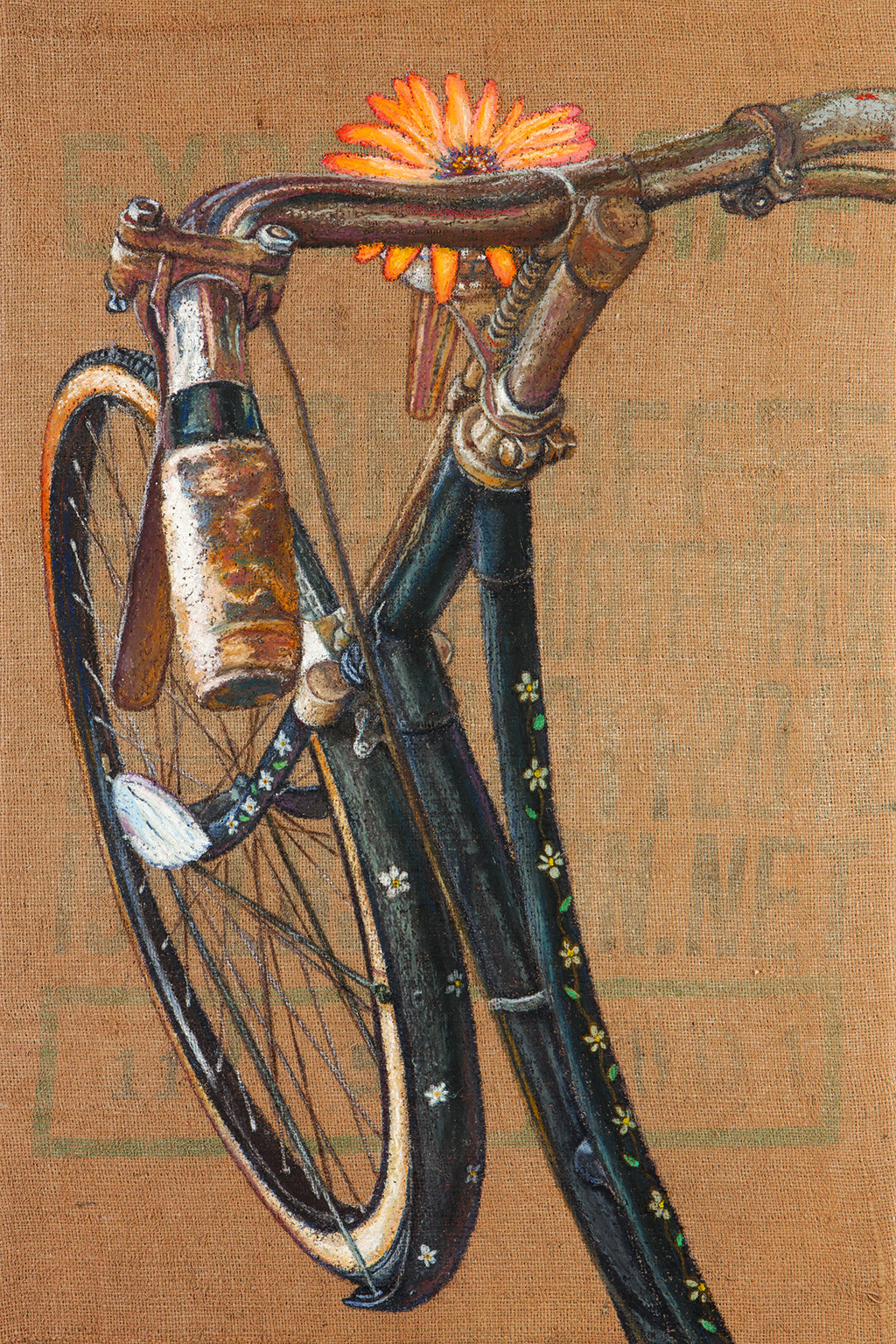This detailed painting captures the front half of an antique-looking bicycle, likely from the late 1800s or early 1900s. The bicycle's frame and handlebars appear to be made of dark, brownish wood rather than the more common modern silver. The background is a textured surface, resembling tan canvas or burlap, with a color similar to an ace bandage.

Prominently featured is the front wheel, which sports more spokes than contemporary bicycles, surrounding a tire with a distinctive white wall. The handlebars, complete with hand brakes, are old and worn, exuding a sense of history. Attached to the front of the handlebars is a small holder containing a single daisy, its bright petals contrasting against the overall dark tones of the handlebar.

The bicycle’s frame, forks, and fenders are painted black, adorned with an intricate and charming pattern of white and yellow flowers interconnected by delicate vines. These painted flowers extend to the poles of the wheels and other metal parts, enhancing the vintage aesthetic of the bike. The entire scene evokes a nostalgic feel, capturing the timeless beauty of an old-fashioned bicycle with detailed and artistic craftsmanship.